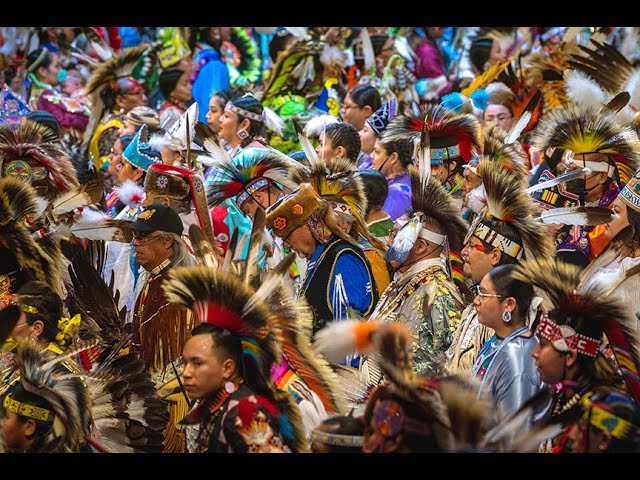This photograph captures a densely packed assembly of First Nation people, with heads and torsos filling the frame. The group consists of men and women, ranging from the young to the elderly, many adorned with intricate, indigenous headpieces embellished with fur, beads, and colorful feathers. The crowd is clothed in a vibrant array of attire, featuring shades of blue and brown as well as a spectrum of colors including red, yellow, black, orange, white, green, neon blue, navy blue, and purple. Some individuals are looking straight ahead, while others have their heads bowed, creating an impression of meditation or prayer. The scene conveys a sense of celebration, with participants wearing ornate and detailed garments, indicating a traditional gathering or ceremony.